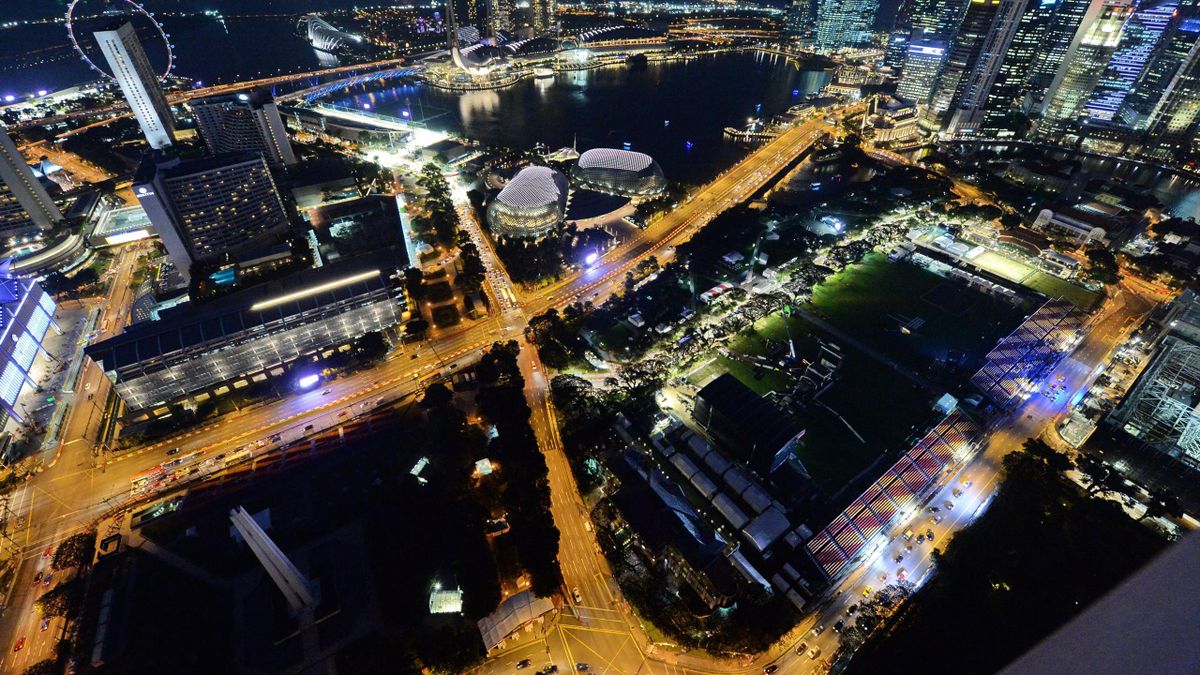This is a captivating aerial photograph of a bustling cityscape at night. The streets, glowing a soft golden-orange from the streetlights, criss-cross the city forming an illuminated X pattern at the center. The well-lit roads highlight intersections and highways, revealing a city vibrantly alive with activity. Surrounding these roads are numerous skyscrapers and tall buildings, their windows shimmering with lights and adding to the city's electrifying ambiance. Towards the middle, there is a rectangular football field, its green barely visible as it's unlit, hinting at its closure for the night. In the upper central part of the image, a sizable body of water can be observed, reflecting the city's luminescence. To the top left stands a brightly lit Ferris wheel, adding a whimsical touch to the urban landscape. The mixture of rectangular and circular buildings displays a dynamic and dense skyline. The scene is void of identifiable signs, focusing instead on the geometric beauty of the lit streets and buildings. Overall, it's a mesmerizing depiction of urban life, captured from above, possibly by a drone, showcasing the intricate layout and vibrant energy of the city at night.